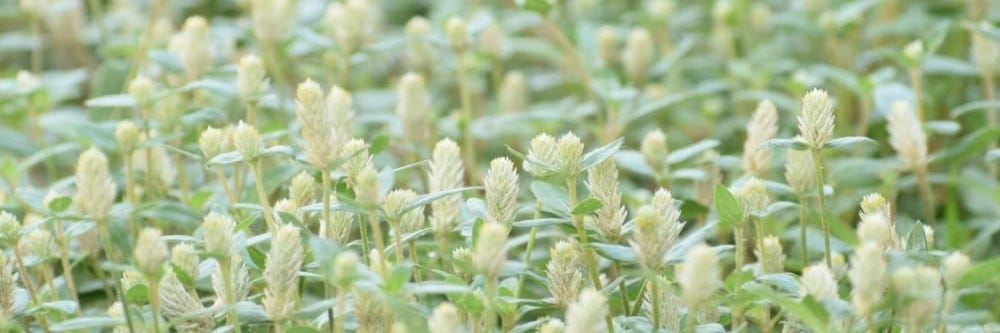This is a close-up photograph of a field dominated by off-white, fluffy, and feathery flowers, likely seed heads, set against a backdrop of light green leaves and stems. The plants have elongated, oval-shaped flower heads resembling rabbit tails, which appear to be illuminated from above. The background is blurred, directing focus onto the greenery and the soft, white floral elements in the foreground. The uniformity and repetition of these plants, with their delicate, vanilla-colored flowers and short, stubby green leaves, create a serene and natural scene that would be ideal for a nature-themed website header or similar use.